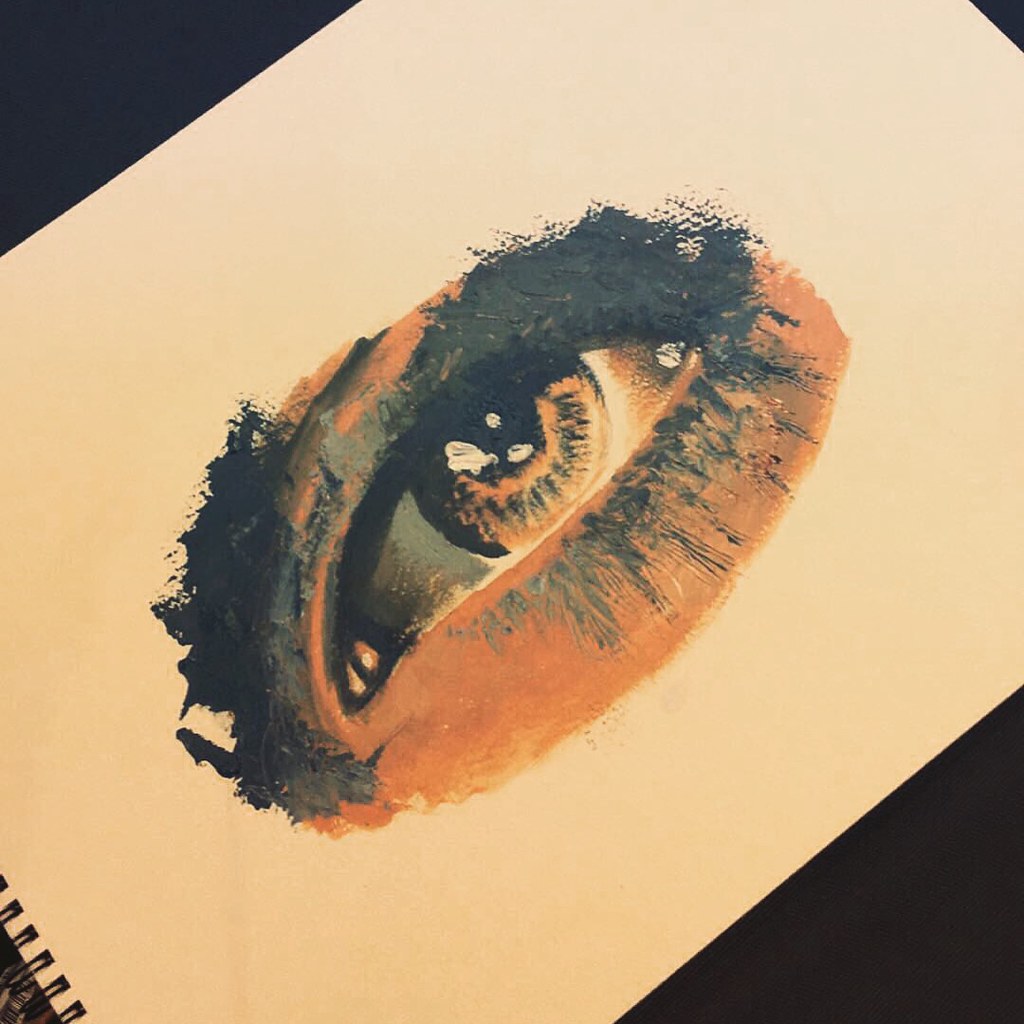This acrylic painting, rendered on slightly off-white paper in a spiral-bound artist's notebook with black spirals, showcases a mesmerizing eye. The eye, painted in rich, deep amber hues, sits against a backdrop of subtly tanned skin. The sclera, or white part of the eye, leans towards an off-white shade, enhancing the naturalistic effect. Embellished with black lashes and a hint of eyebrow detail, the eye's lower lid features a noticeable white highlight, adding depth and realism. The lower eyelashes are prominently visible, adding texture, while the upper eyelashes are more softly blended, giving the eye a compelling, mottled appearance. The four corners of the image are artfully darkened, framing the eye and drawing the viewer's focus inward.